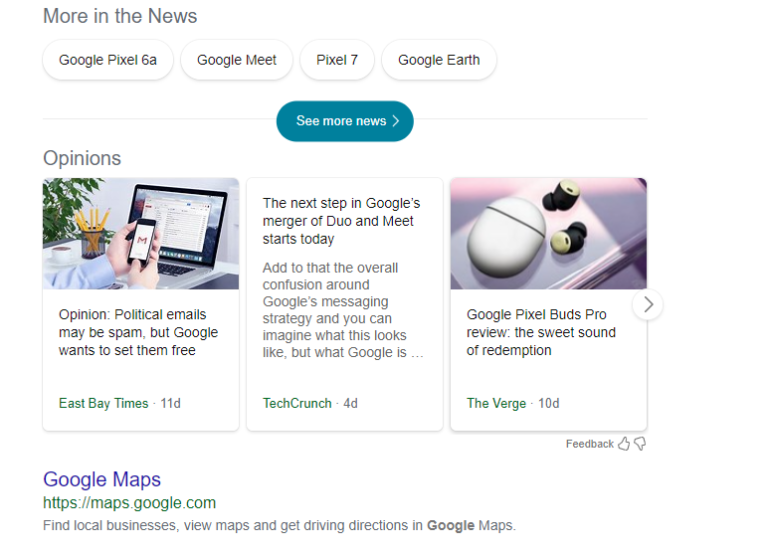The image depicts a Google search page with an array of information. At the top left, there is a section labeled "More in the News." Directly below this heading are four oval buttons. The first button on the left reads "Google Pixel 6a," followed by "Google Meet" to its right, a button labeled "Pixel 7" adjacent to that, and "Google Earth" as the final button. 

Centered underneath these buttons is a blue, oval-shaped button labeled "See more news," distinguished with a right-pointing arrow inside it. Below this button on the left side is the section "Opinions." Here, it displays an article titled "Opinion: Political emails may be spam, but Google wants to set them free," accompanied by a media image of someone holding a phone and looking at their laptop. This article is attributed to "East Bay Times."

Next to this, another section presents an article about the merging of Google's Duo and Meet services, indicating this integration begins today. Adjacent to this article is a review titled "Google Pixel Buds Pro Review: The Sweet Sound of Redemption," featuring a computer-generated image of the Pixel Buds Pro.

Towards the bottom of the page, there is a highlighted section for "Google Maps," highlighted in blue, with the HTTPS web address prominently displayed. Beneath this, there is a description offering functionalities such as finding local businesses, viewing maps, and getting driving directions via Google Maps.